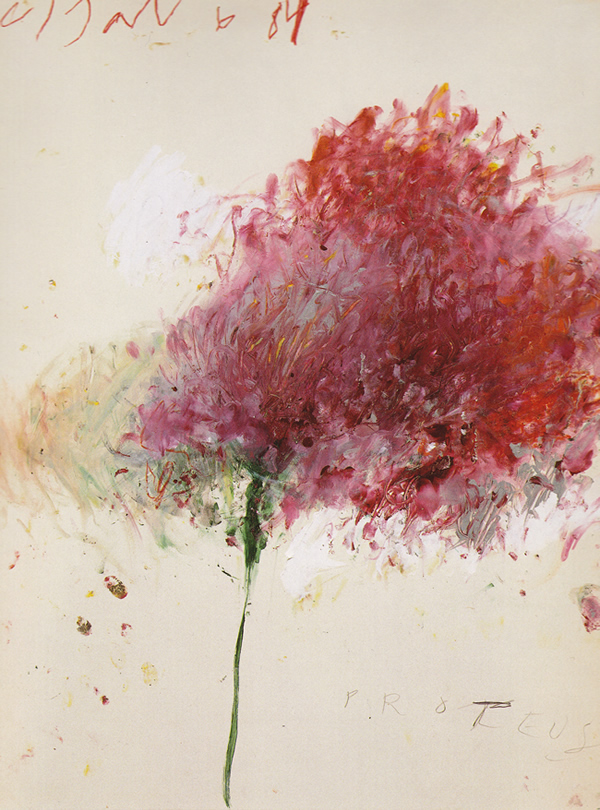This image is an abstract painting on white paper, dated 1984, as suggested by the scraggly signature and the number "84" in the top left corner. At the bottom, "Proteus" is crudely written in pencil. Dominating the composition is a powerful, chaotic depiction of a flower, primarily characterized by a large splotch of reddish pink that occupies almost a third of the painting. The brushstrokes appear hurried and energized, especially on the right side where the red and pink hues are the most intense, interspersed with touches of orange and yellow. Contrary to this, the left side of the flower appears incomplete, with disintegrating brushstrokes in light tan and green hues. A dark green, thin stem extends to the bottom center of the image, grounding the abstract petals that seem to be blowing to the right, as if caught in a breath of wind. Small bits of white and other subtle details emerge upon closer inspection, lending a complex, almost floral effect to the overall composition amidst the off-color white background.